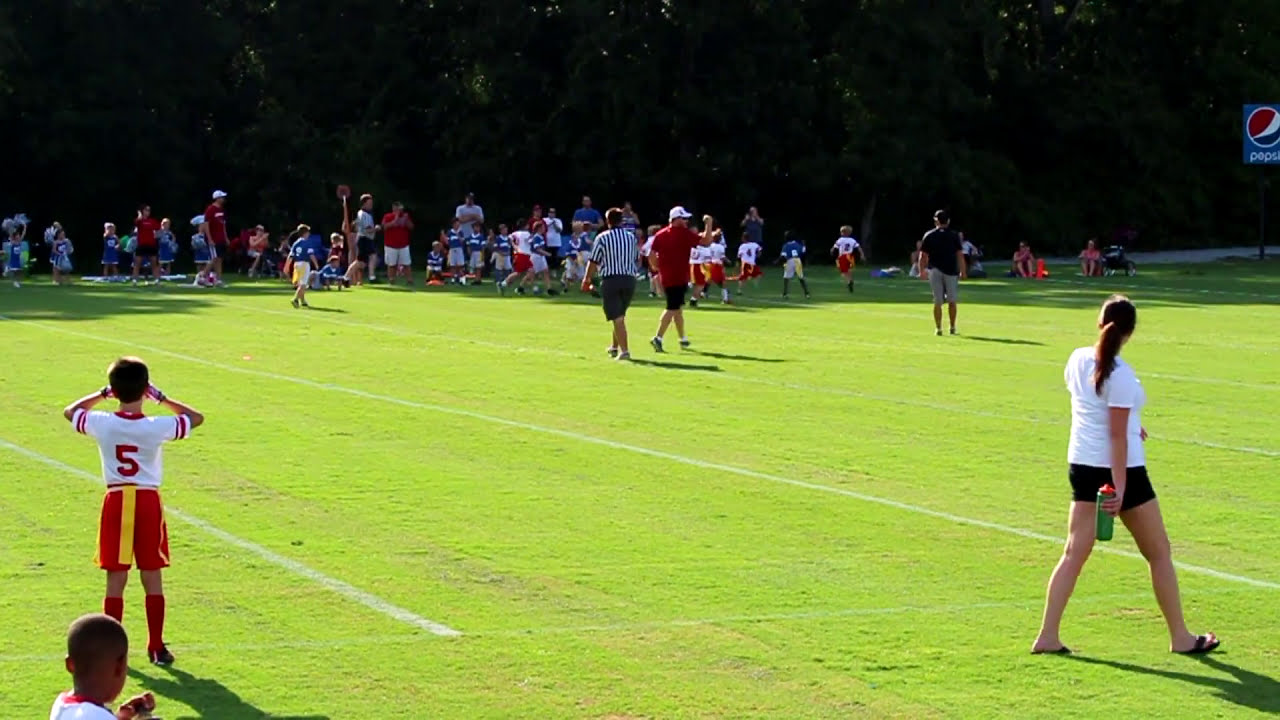The image captures a lively scene on a kid's soccer field during a bright, sunny day, surrounded by tall, dark green trees in the background. The central focus is on the referee wearing a black and white striped shirt and black shorts, standing slightly above the center of the frame. To the referee’s right, a coach in a white hat and red shirt is visible, while another coach, partially balding and dark-skinned, is seen walking towards the center from the right side of the field.

In the bottom left corner, two children are noticeable: one in a white shirt with a number 5 on his back, red pants, and a yellow belt, and another slightly balding, darker-skinned kid. Most children are with the adults seated or standing in the background, positioned primarily behind and to the left of the referee. The playing field has a mixture of yellowing grass with white strips marking the boundaries, angled from the bottom left of the frame towards the seated crowd. Additionally, the scene includes various details like a bench, little cheerleaders, and a scoreboard with the Pepsi logo, showcasing a structured setting indicative of a regulated game, likely flag football, played by boys around 8 to 10 years old, wearing different colored team uniforms.